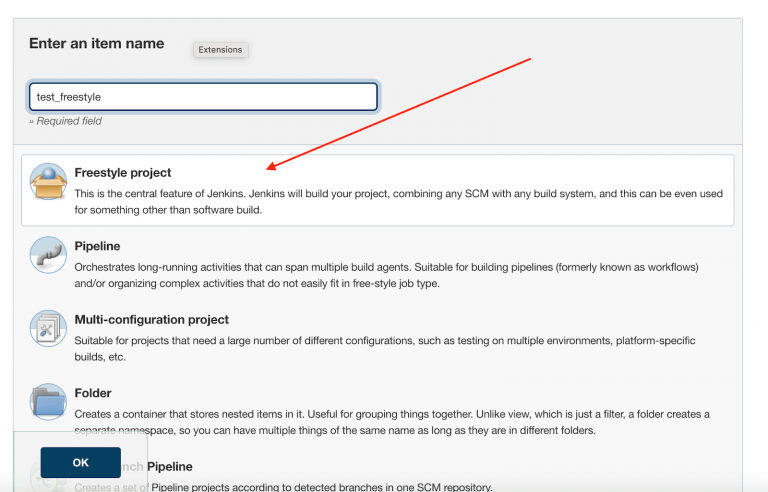A screenshot taken from a computer displays a Jenkins interface. In the center of the image, there is a text field prompting users to "Enter an item name," in which "test_freestyle" has been input. Consequently, "Freestyle Project" has appeared below this field. 

A thin, red arrow extends from the top right corner of the screen, pointing downwards towards the "Freestyle Project" option. This section is illuminated by a description highlighting its significance: "This is the central feature of Jenkins. Jenkins will build your project combining any SCM with any build system. This can even be used for something other than software builds."

Below the "Freestyle Project" selection, additional options are listed, including "Pipeline," "Multi-configuration project," "Folder," and "Launch Pipeline." Over the "Launch Pipeline" section, a navy blue 'OK' button with white text is prominently displayed. 

The description for the "Pipeline" option elaborates on its function: "Orchestrates long-running activities that can span multiple build agents. Suitable for building pipelines, formerly known as workflows, and organizing complex activities that do not easily fit in freestyle job types." 

The lower portion of the screen is partially cut off, hinting at additional details about the "Launch Pipeline" feature.